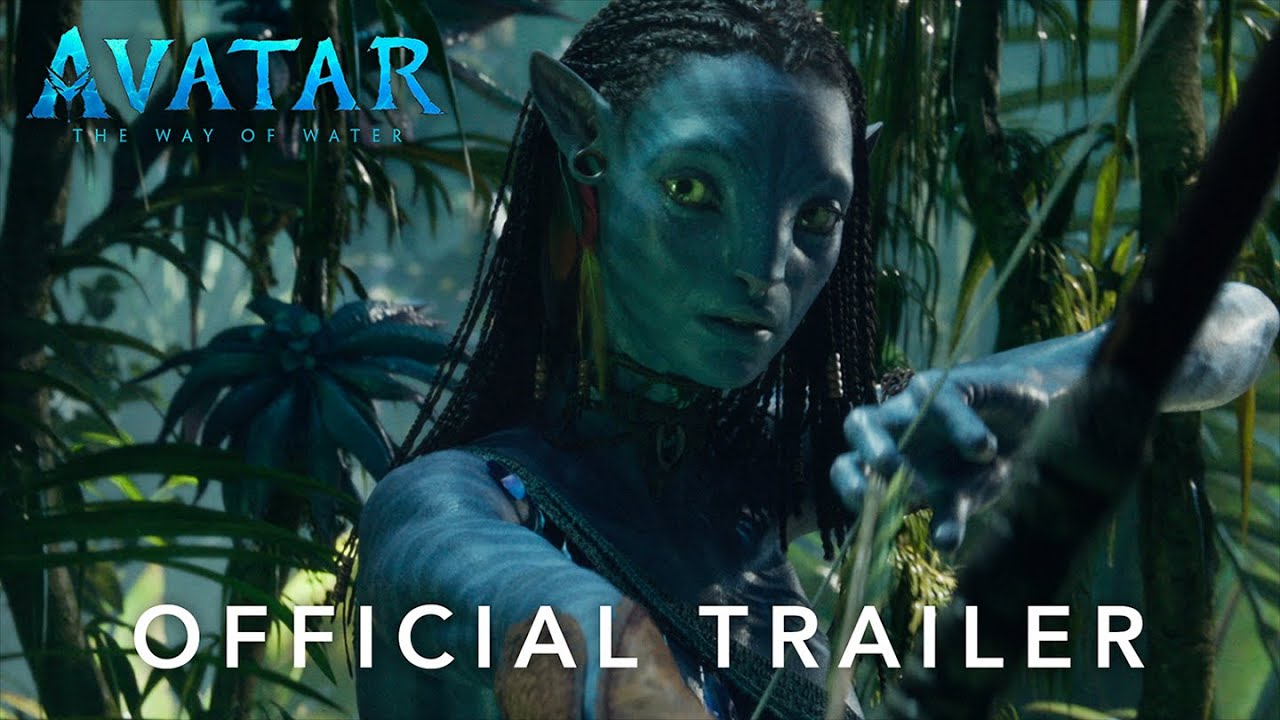This image is an official poster for the movie "Avatar: The Way of Water." It prominently features a blue-skinned, alien creature with distinct humanoid and feline characteristics. The character's face is mostly human-like but with more widely spaced, cat-shaped yellow eyes, and pointed ears positioned towards the top of the head. She has long, braided black hair adorned with earrings, and her skin is patterned with blue tiger-like stripes. The character is depicted in a lush, tropical jungle setting, with different shades of greenery and various trees in the background. She is seen with her left arm resting against a tree, staring intently at the viewer. The poster includes text at the top left in blue letters reading "Avatar: The Way of Water," while the bottom displays "OFFICIAL TRAILER" in white capital letters. This detailed portrayal underscores the exotic and immersive environment of the movie, as well as highlights the character's intricate and otherworldly design.